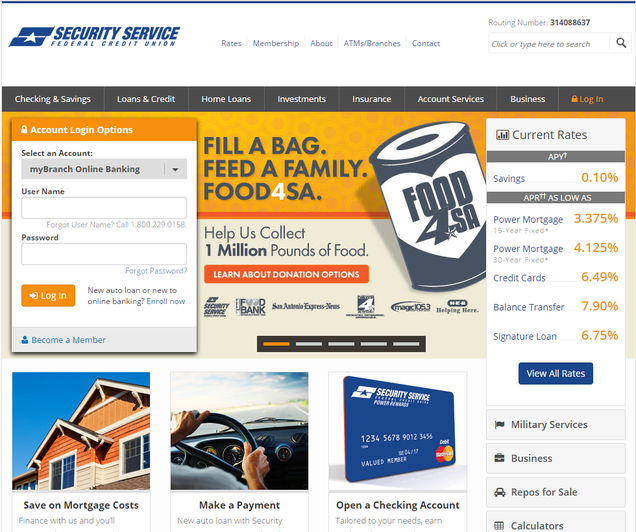The website likely belongs to Security Service Federal Credit Union. The top left corner features their name and logo, with "Security Service Federal Credit Union" written in all caps. "Security Service" is presented in a larger, bold font. A banner stretches across the top of the page, containing five clickable links: "Rates," "Membership," "About," "ATM/Branches," and "Contact."

In the top right corner, there's a label indicating the "Routing Number," specifically 314088637. Below this, a search input field prompts users with the text "Click or type here to search," accompanied by a search icon.

The main content showcases a prominent message in the center: "Fill a Bag, Feed a Family, Food #4SA." Beneath this, the text encourages participation with the call to action, "Help us collect 1 million pounds of food."